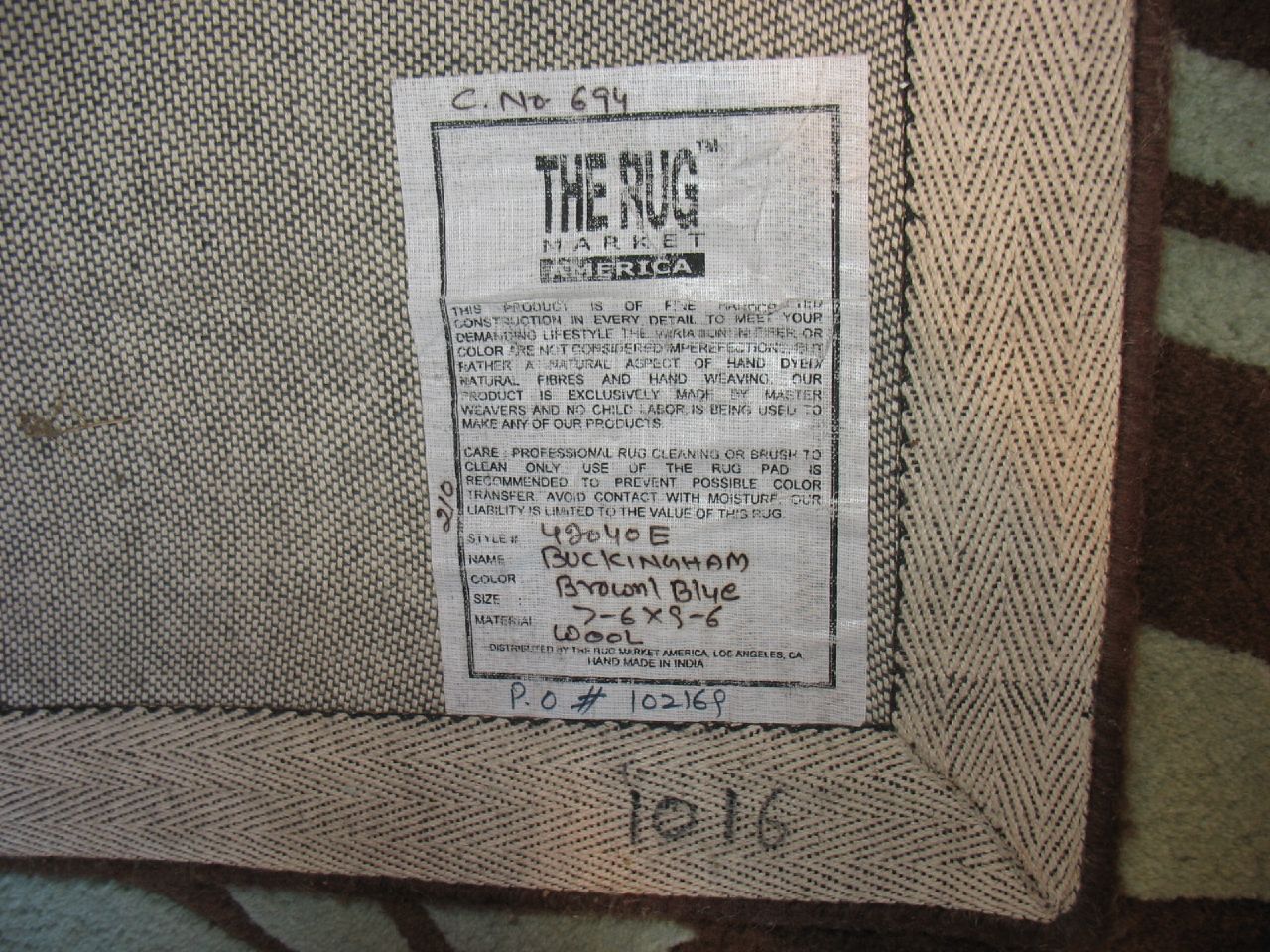This photograph captures the underside of a rug, showcasing a detailed label from The Rug Market America. The tan and black squares on the rug’s back transition into diagonal patterns along the edge, with brown and white stripes of varying thickness positioned to the right. A white label, bordered in black, is affixed to the rug and features black handwritten text. The label prominently states the style number as 42040E, the rug’s name as Buckingham, and indicates the color is brown/blue. The woolen rug, measuring 7'6'' by 9'6'', is handmade in India and distributed by The Rug Market America in Los Angeles, California. Notes on the label emphasize that the product is crafted by master weavers without the use of child labor. It advises professional rug cleaning, the use of a rug pad to prevent color transfer, and warns about liability limited to the rug's value. Additional faded text mentions the natural aspect and fine construction, ensuring durability to meet demanding lifestyles. The photograph is landscape-oriented, highlighting the corner and details of the rug.